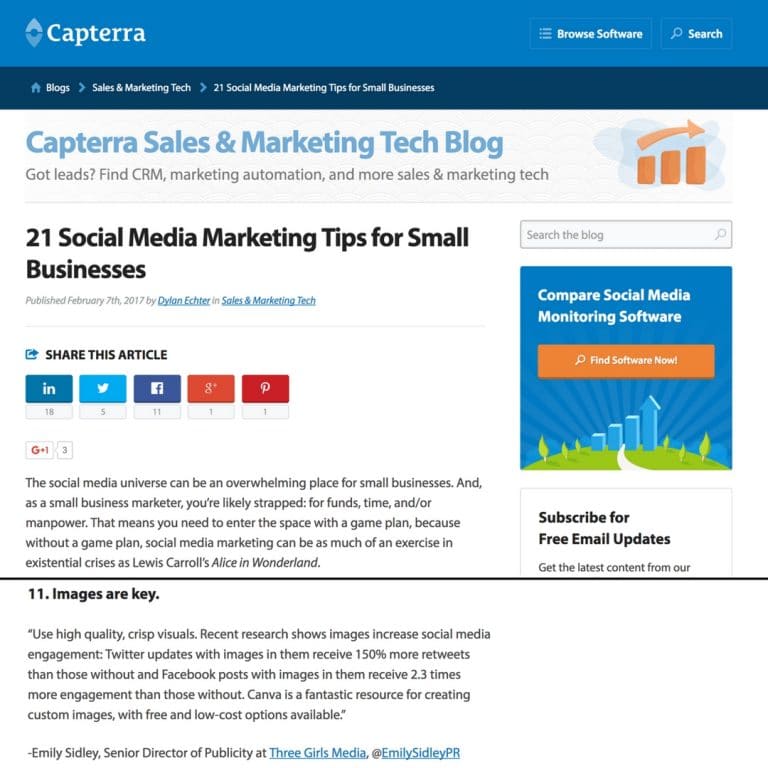This detailed caption accurately and comprehensively describes the image:

"A colorful square-format screenshot of a webpage from the company Capterra, featuring its logo on the left that consists of a simple up-and-down arrow symbol. The company name, 'Capterra', is styled with a capital 'C' followed by lowercase letters. The webpage has a light blue banner at the top, followed by a slightly darker blue banner below it. This darker banner contains tabs for navigating to various sections, including 'Blogs,' 'Sales and Marketing Tech,' and an article titled '21 Social Media Marketing Tips for Small Businesses.'

The main focus of the screenshot is this article, prominently displayed with a bold black headline announcing '21 Social Media Marketing Tips for Small Businesses.' Authored by Dylan Escher, the article is dated February 7, 2017. Readers have the option to share the article via LinkedIn, Twitter, Facebook, Google, or Pinterest. On the right-hand side of the webpage, there's a feature inviting visitors to 'subscribe for free email updates.' The screenshot, effectively a front page or inner page of the Capterra website, provides a glimpse into the company's online content and layout."